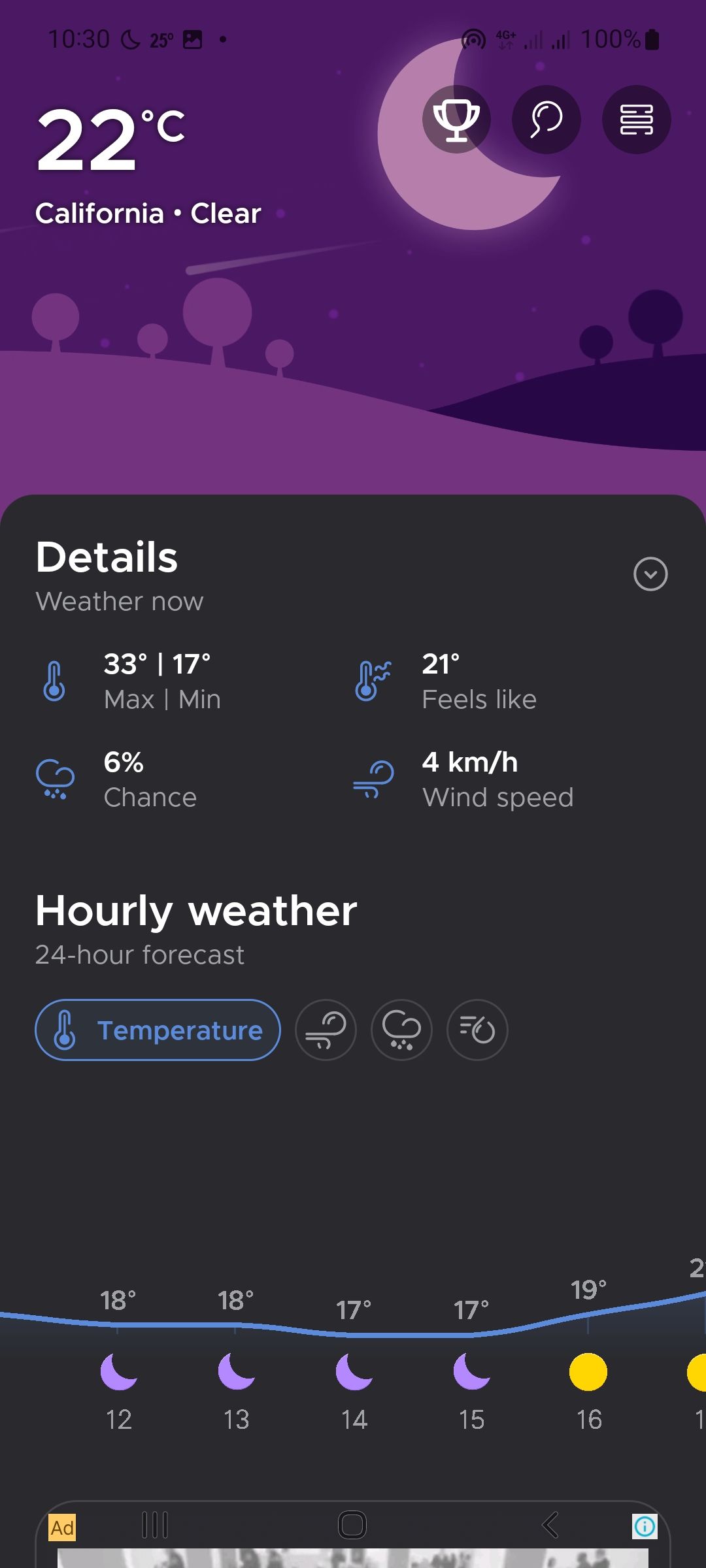This image depicts a home phone screen showcasing a California weather forecast. At the top of the screen, there is a purple background with faint cell phone icons, making them hard to discern. The time displayed is 10:30, and the battery percentage is at 100%, located on the right side. The backdrop features a crescent moon and simple illustrations of trees and hills. In the top section, it indicates the temperature is 22 degrees Celsius with clear weather conditions in white text to the left. Adjacent to this are a trophy icon, a search icon, and a white square icon aligned to the right.

Beneath this section, the word "Details" is prominently displayed in white, followed by "Weather Now" in gray. This area provides four specific weather metrics: a maximum temperature of 33 degrees Celsius, a minimum of 17 degrees Celsius, a 6% chance of rain, a "feels like" temperature of 21 degrees Celsius, and wind speeds of 4 km/h.

Further down, the screen offers an hourly weather prediction and a 24-hour forecast, marked by a blue tab indicating temperature, with three accompanying icons on the right. Under this section, a light blue line is present with numerical values positioned above and below it. Among these icons, the first four depict a light purple moon, while the two icons to the right are represented by a yellow circle. At the bottom, part of an advertisement is visible, set against a black background.